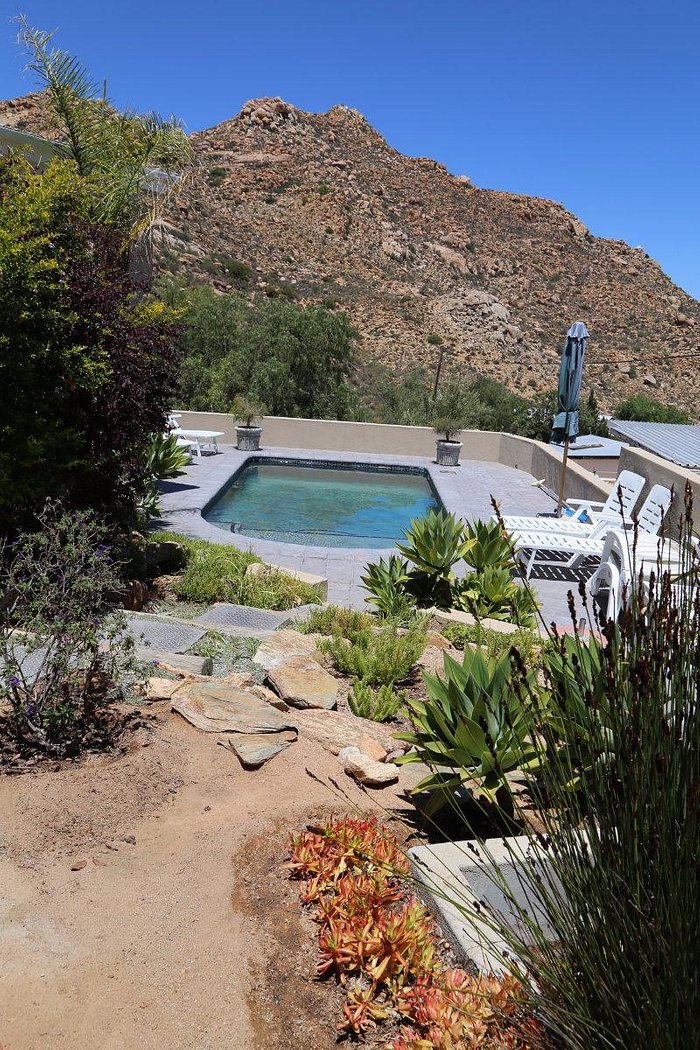This image captures a serene backyard pool setting amidst a rustic landscape. At the center, a small, bluish-green pool is encircled by a paved deck featuring patio furniture, including several white lounge chairs and a folded blue umbrella on the right side. Additional lounge chairs are partially concealed by a tree in the back left corner, and two green potted plants are positioned at the very back corners of the pool. The surrounding area showcases a mix of greenery, including tall shrubs and succulents, indicating a desert-like environment. A dirt path leads to this cozy pool area, which is framed by a sizable, dusty hill or small mountain covered in brown, rocky sediment, enhancing the picturesque view. This idyllic poolside retreat, likely set in a Midwestern or Californian locale, offers a blend of natural beauty and inviting relaxation.